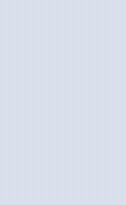The image displays a vertically oriented rectangle, approximately twice as long as it is wide, featuring a simple white background with a gradient transitioning through shades of blue and black. A thin yellow border frames the rectangle, which also contains a central band of a tannish yellow color.

Down the left side of the image, a series of icons paired with text provide guidelines for interpreting visual elements:
1. A yellow-bordered box at the top contains the phrase "Think about." Directly below, an image icon appears with the text: "What is the image on first glance?"
2. Below the image icon, a light bulb with a yellow top and a blue screw bottom accompanies the text: "What are the objects and their counts?"
3. Further down, there's an icon of a piece of paper and pencil with the text: "What does the text say?"
4. Next, a red pen pointing downward accompanies the text: "What are the positions of the objects?"
5. Below the pen, a magnifying glass with its handle directed downward to the left includes the text: "What subtle details are noticeable?"
6. Further down, a stylized building with a blue top and gray sides, standing three to four stories tall, is paired with the text: "What is in the background?"
7. Lastly, a green circle is accompanied by the text: "What is the style and color?"

Black dots are positioned to the left of each icon, creating a cohesive visual guide along the left side of the image.